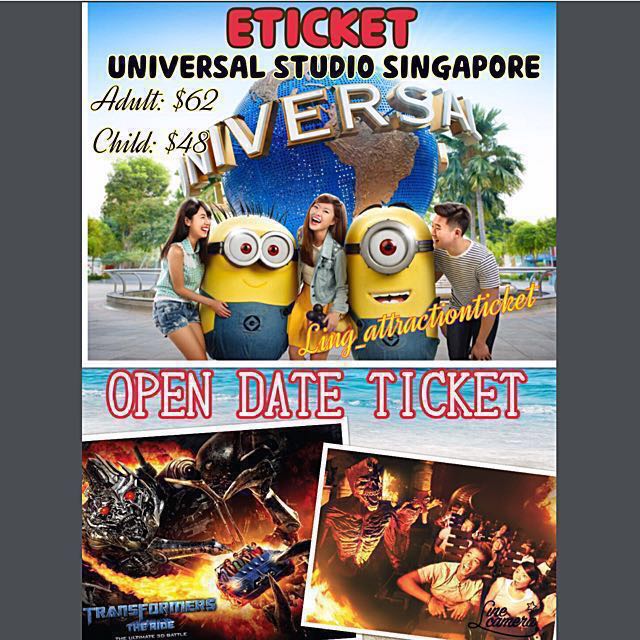**Photo 1**: 

A vibrant digital poster from Universal Studios Singapore showcases the iconic entrance of the amusement park. Central to the image is the famous rotating globe fountain, emblazoned with "Universal" in bold letters. Posed cheerfully in front of the globe are three Asian visitors - two females and one male. The female on the left and the male on the right flank a Minion character, while the woman in the middle adds to the jovial scene. In the lower right corner of the image, a slanted banner reads "Ling Attraction Ticket," while the top right corner details the pricing: "Adults: $62" and "Child: $48." Just above the Universal Studios Singapore logo, "e-ticket" is prominently displayed. 

**Photo 2**:

The lower section of the poster promotes a "One Day Ticket" and features two dramatic movie-poster-like images of popular rides at the park. The first image appears to be themed around either "Back to the Future" or "The Mummy," while the second depicts the thrilling "Transformers" ride. Both poster images are action-packed and ablaze with flames, adding to the dynamic and exciting appeal of the attractions.